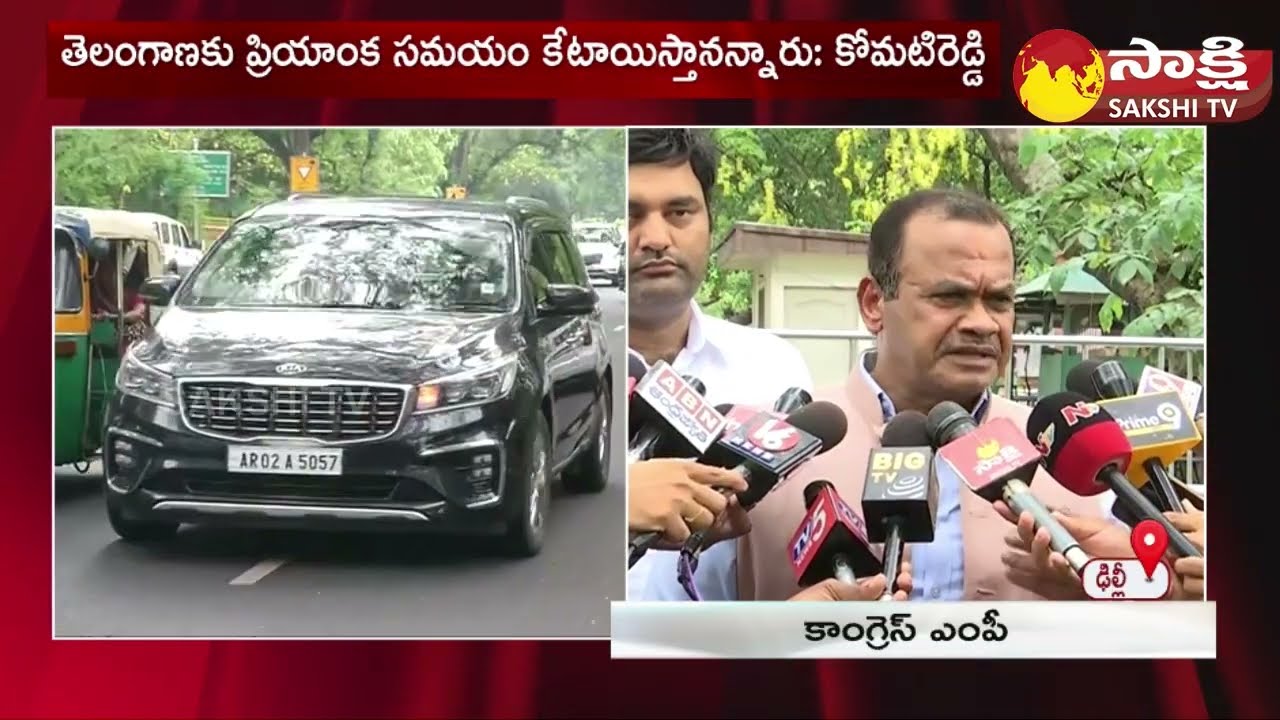This image appears to be a screenshot from an East Indian news broadcast on Sakshi TV, characterized by its red-bordered split-screen layout. On the left side, a dark grey to black minivan with an Indian license plate, AR02A5057, is prominently displayed. Above the vehicle, white script in Indian writing stretches across the top of the screen. The right side of the screen features a middle-aged, brown-skinned man in a pastel-colored jacket and blue shirt, speaking to reporters. This man is captured mid-speech, squinting slightly and frowning, with eight microphones from various TV stations thrust in front of him. Behind him, another man stands, gazing blankly at the reporters. The top-right corner of the screen includes the Sakshi TV logo, a circular emblem resembling a globe in yellow and red, with additional Indian script next to it. The overall scene is quintessential of a news program setup, providing a vivid glimpse into the bustling atmosphere of a live news interview.